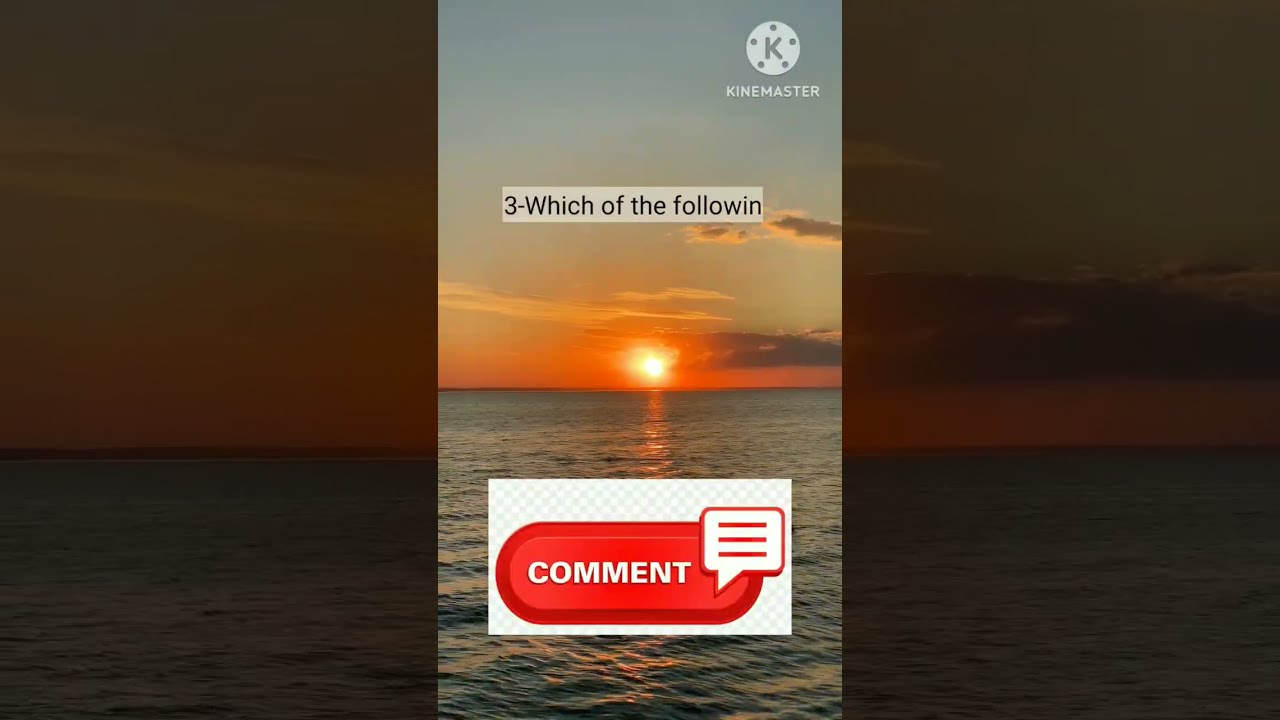This image captures a serene sunset over a vast, ripple-kissed ocean with no visible landmarks in sight. The sky transitions from deep reds and oranges near the horizon to a lighter blue as it ascends, punctuated by some white and gray clouds that do not obstruct the view of the setting sun. Overlaid on this tranquil scene, the top right corner features the KineMaster logo, a see-through "K" inside a white circle bordered by five dots, with "KINE MASTER" written underneath. The central portion of the image displays a text box with "3-WHICH OF THE FOLLOWING" in black letters on a white background. Towards the bottom, a prominent red comment button featuring white text and a speech bubble icon hovers over the water. The overall atmosphere exudes stillness and natural beauty, accentuated by the unobstructed horizon and vivid colors of the retreating day.